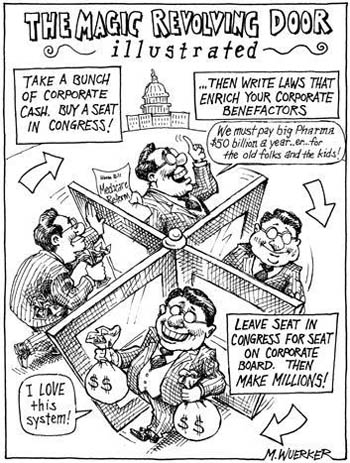This black-and-white political cartoon titled "The Magic Revolving Door Illustrated" conveys a critical commentary on the corrupt relationship between corporate money and politics. The central figure, depicted in an old-school, cross-hatched art style, is shown repeatedly entering and exiting a revolving door, symbolizing the cycle of corruption. The captions narrate his journey: "Take a bunch of corporate cash, buy a seat in Congress, then write laws that enrich your corporate benefactors." Another panel features the character stating, "We must pay Big Pharma $50 billion a year for the old folks and the kids." As he exits the revolving door, the text reads, "Leave seat in Congress for a seat on corporate board, then make millions," with the character exclaiming, "I love this system," while clutching bags full of money. The background includes a black outline of Capitol Hill, emphasizing the connection to Congress, and illustrative arrows emphasize the repetitive, cyclical nature of this corrupt system.